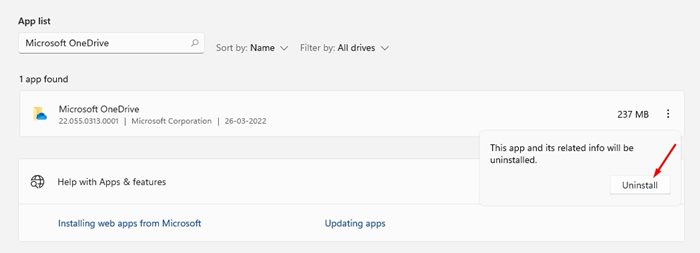The image features a user interface set against a light gray background. At the upper left corner are the words "AppList" in black letters. Directly below is a search bar containing the text "Microsoft OneDrive." Adjacent to the search bar, there are two dropdown options: "Sort by name" and "Filter by all drives," both indicated by downward-pointing arrows.

Beneath these dropdowns, a text line reads "1 app found" in black. Following this, there's a detailed listing of the app, displayed against a white background. The app is identified as "Microsoft OneDrive" with version 22.055.0313.0001, published by Microsoft Corporation on 26-03-2022. To the right of this app description, there's a file size indication of "237 MB," accompanied by a vertical ellipsis (three dots).

Further down, there is another white rectangular section stating "Help with apps and features." To its right, a message reads "This app and its related info will be uninstalled," which points to a red 'Uninstall' button.

At the bottom of the image, in blue letters, it says "Installing web apps from Microsoft," and directly to its right, also in blue, is the text "Updating apps."